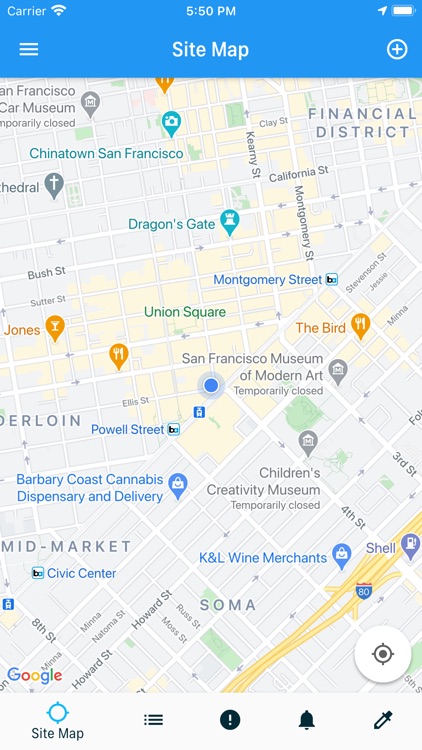The image is a detailed screenshot from Google Maps, showcasing a section of San Francisco. At the top, the interface displays a dark blue bezel. To the left, the status indicates "carrier" accompanied by a wireless symbol, and three horizontal lines that presumably lead to settings. The current time is 5:50 PM, displayed prominently in the center, with "site map" written in bold white below it. On the top right, an arrow pointing to the right and a nearly full battery icon are visible, beside a circle containing a plus sign.

The central part of the image is dominated by the map, populated with various labels and icons. On the right-hand side, the map highlights the "Financial District" in dark grey. Towards the middle, the "San Francisco Museum of Modern Art" is marked, noted as "temporarily closed," with a museum symbol next to it. Below, the "Children's Creativity Museum" also appears, similarly marked as "temporarily closed."

Several points of interest are indicated by various pins:
- A blue pin with a shopping bag icon marks the "Barbary Coast Cannabis Dispensary and Delivery" to the left.
- Near Interstate 80, a shield in blue and red, the "K&L Wine Merchants" is labeled.
- Near the highway, a purple pin with a gas station pump icon indicates a nearby Shell gas station.

The area also features several dining locations:
- On the far left, partially cut off, a wine glass pin marks a place named "Jones."
- Beneath "Montgomery's Sheet" (a cyan square pin), "The Bird" is marked with an orange pin depicting a fork and knife.

Additional icons include:
- A cyan blue camera pin marking "Chinatown San Francisco."
- The "San Francisco Car Museum" labeled on the left.
- A church or cathedral is also noted to the left.
- "Dragon's Gate" is highlighted with a cyan blue pin featuring a white chess piece icon.

The map section is a snapshot rich in detail, offering insight into the various cultural, commercial, and service-oriented locations within San Francisco, some of which are temporarily closed.